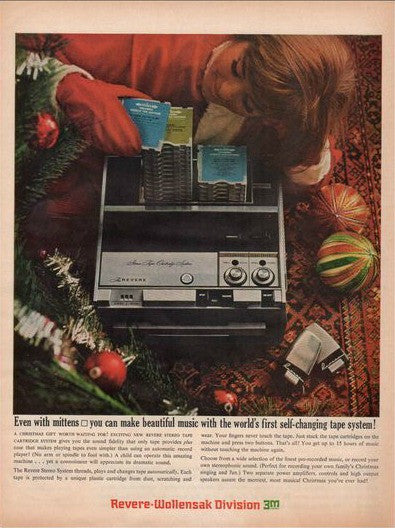The advertisement from a vintage magazine, likely from the 1970s or 1980s, features a scene set during Christmas. Central to the image is a silver cassette player with a black top, adorned with various dials and buttons. A stack of cassette tapes rests on top of the player. A woman with dark hair and bangs, wearing red mittens and a red shirt, is seen leaning or laying on an oriental rug under a Christmas tree, which is decorated with tinsel and red balls. Scattered around her and the tape player are colorful Christmas ornaments in green, red, and white. The text on the ad reads, "Even with mittens you can make beautiful music with the world's first self-changing tape system." Additional small print follows this declaration, though it is difficult to read, and at the bottom, bold red text states, "Revere-Walensak Division of 3M."